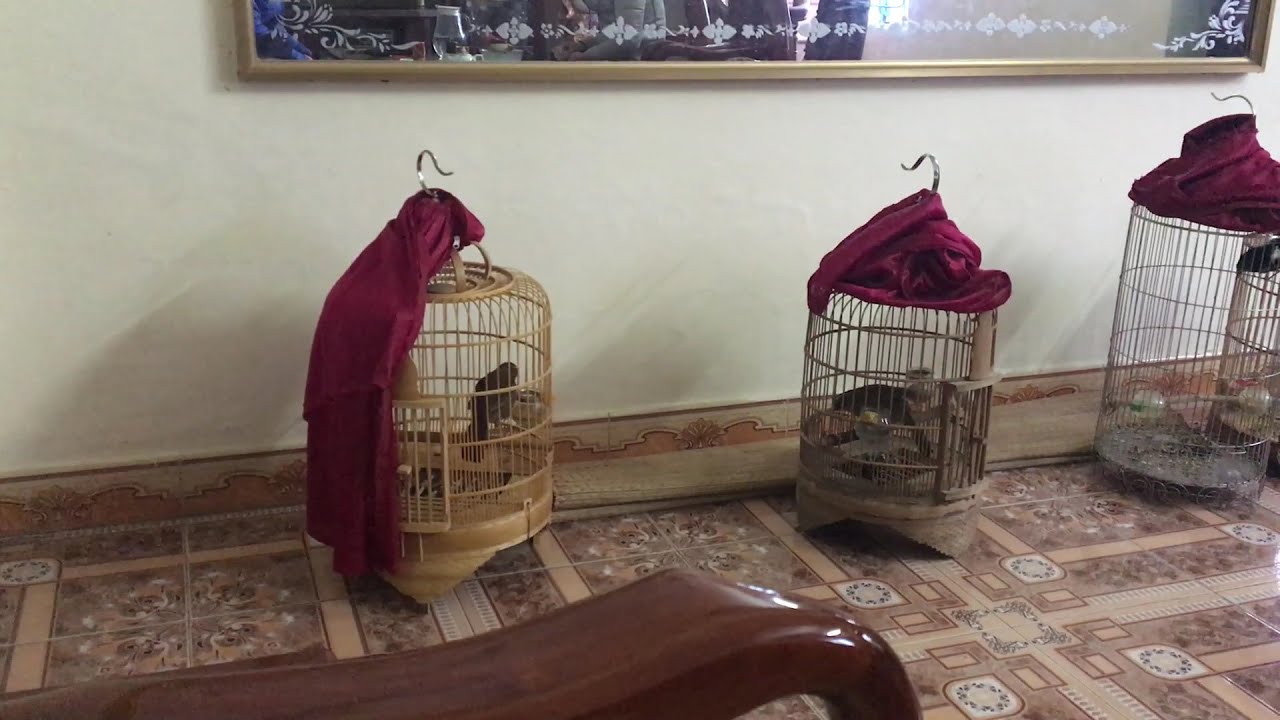In an elegant, historic room with intricately tiled parquet floors and ornate baseboards leading up to solid cream-colored walls, three birdcages are arranged in a row, each spaced about a foot and a half apart. The cages, which vary in color from golden brown to dark brown to metallic gray, house birds within their confines. Each cage is adorned with a maroon drape cloth that is partially pulled back to reveal the birds inside. The tops of the cages feature gold hooks. Above the cages, a large, decorative wall mirror with a white-framed edge reflects the room’s timeless charm. In the lower left corner of the image, the curved arm of a wooden chair subtly enters the scene, adding to the room's vintage ambiance.